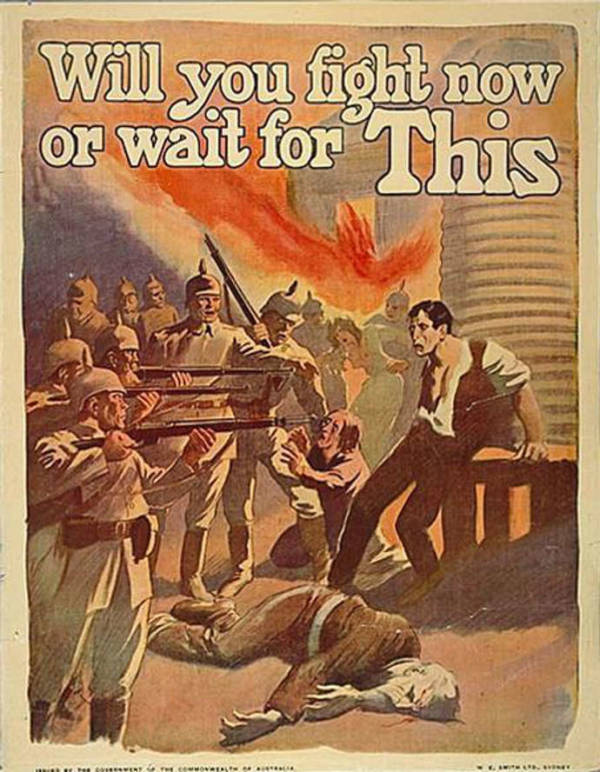The illustration, bordered by a tan-yellow frame, is a vintage-style poster featuring a dramatic and intense scene. At the top, in bold tan-yellow text surrounded by a black and white border, reads, "Will you fight now or wait for this?" Dominating the foreground, several soldiers dressed in tan uniforms including black belts, boots, and spiked helmets, aim their rifles at a distressed man, who, with a torn white shirt and brown pants, leans backwards in despair against a bench on the right side. Beside him, a woman kneels, pleading with the soldiers. Another man lies dead on the ground, adding to the scene's gravity. In the background, a town is ablaze, and a solitary silo stands ominously to the right, accentuating the chaos. The soldiers’ commander, distinguishable by his authoritative stance and raised baton, directs the violent tableau. This powerful image evokes a call to action, compelling the viewer to consider the choice between fighting now or facing a dire fate later.